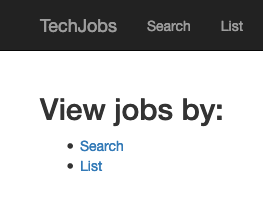The webpage displayed is a job search platform titled "Tech Jobs." The top header, which is black with gray text, prominently features the site's name on the top left. Adjacent to the name, towards the right side of the header, are navigational options labeled "Search" and "List."

Beneath the header, the main page has a clean white background with text primarily in black, and some in blue for emphasis and interaction. At the top of this section, there is a heading in black text that reads "View Jobs By." Below this heading are two bullet points, both featuring blue text that acts as clickable links. The first bullet point says "Search," and the second says "List."

Each of these blue bullet points provides a functional URL: clicking on "Search" takes the user to the search feature, while clicking on "List" directs the user to a comprehensive list of job postings. This setup clearly indicates that users can filter and explore job opportunities based on their preferred method – either through a search function or viewing a list. Overall, the layout is designed to facilitate easy navigation and a straightforward job search experience.